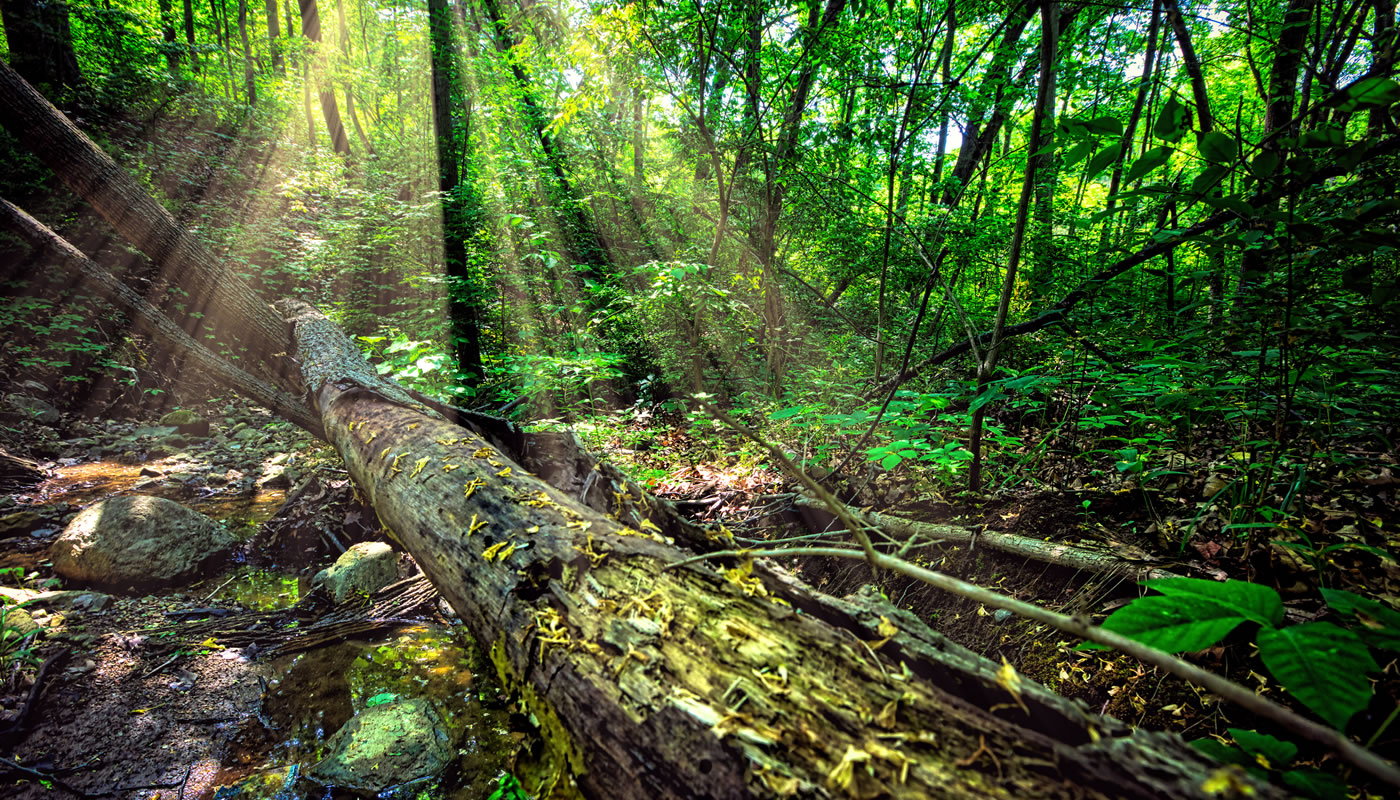In this detailed photograph of a dense forest scene, a large, half-rotten fallen tree commands the foreground, its bark peeling and trunk splitting as it breaks apart. Surrounding the fallen tree, a lush carpet of foliage, small plants, and scattered branches mix with a few prominent rocks, contributing to the rich texture of the forest floor. The background showcases a dense array of green trees, creating an almost rainforest-like atmosphere. Sun rays dramatically pierce through the dense canopy from the left side of the image, bathing the fallen tree and surrounding vegetation in a warm glow, highlighting the scene's natural beauty. A glimpse of blue sky is visible through the treetops, hinting at a sunny day, while a small creek meanders beneath the log, enhancing the photograph’s serene, untouched ambiance.